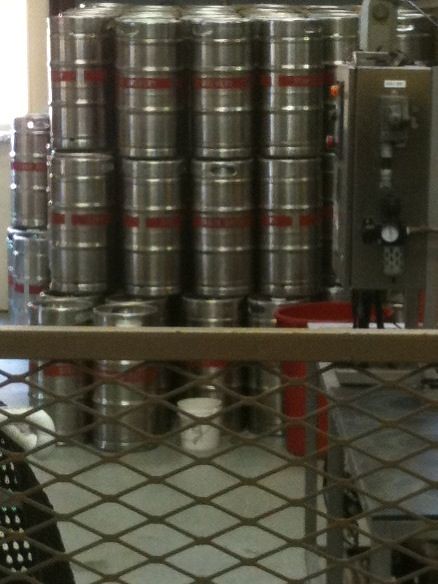The colour photograph showcases a room filled with stacks of tall, slender, cylindrical kegs, each characterized by their dark metallic sheen and distinct red stripe around the center. These kegs are neatly arranged in rows, some stacks reaching up to the ceiling. A notable red bin is positioned toward the bottom of the kegs, almost matching their size. The muted colours of the photo, possibly due to age or a greenish filter, add a vintage feel to the scene.

In the far background on the left, a small portion of a window is visible in the top left corner, with a thin strip of white wall adjacent to it. In front of this wall, two of the kegs are stacked atop each other, echoing the silver and red motif. Further to the right, rows of kegs stand three high, a uniform line of red stripes marking each row. 

The foreground features a distinctive wooden fence with a triangular grid pattern, suggesting the viewer is positioned behind this barrier. Beneath this fence is a ledge in a dark brown hue and a netting structure. A gray steel bar runs across the bottom of the image, underlined by gray fencing, reinforcing the industrial ambiance. 

To the right, beyond the kegs and fencing, a piece of gray machinery equipped with various knobs, levers, and buttons is present, adding to the complexity of the setting. The flooring throughout is light gray, contrasting with the metallic and wooden elements. Overall, the image provides a detailed glimpse into a storage area populated by numerous kegs and industrial fixtures.